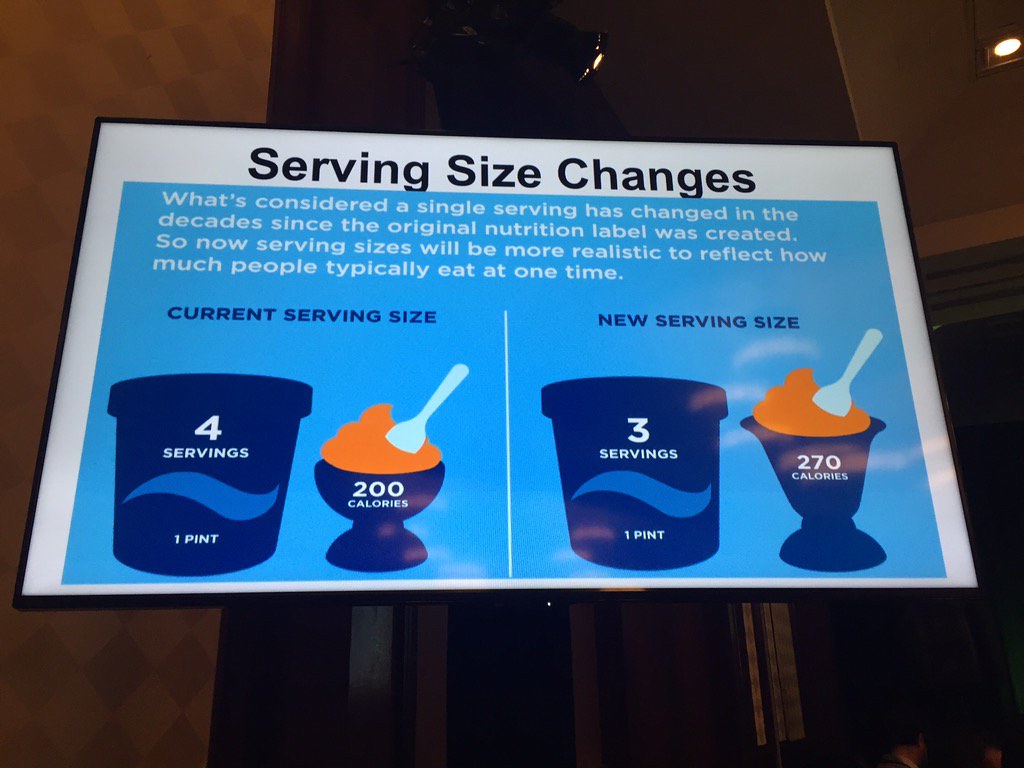Set against a brown table adorned with a few placemats, this rectangular image features a detailed label. This label, framed by a white border and centered on a light blue background, addresses changes in serving sizes. The top of the white border reads, "Serving Size Changes." Against the blue background, the label elaborates that serving sizes have been updated to be more realistic, reflecting the amount people typically consume at one time. 

An illustrative example showcases a pint of what appears to be ice cream. Originally, the container was marked as four servings, with each serving containing 200 calories, depicted by an orange product in a bowl with a white spoon. To the right of this, the label indicates the updated serving size, showing that the container now realistically contains three servings, with each serving being 270 calories.